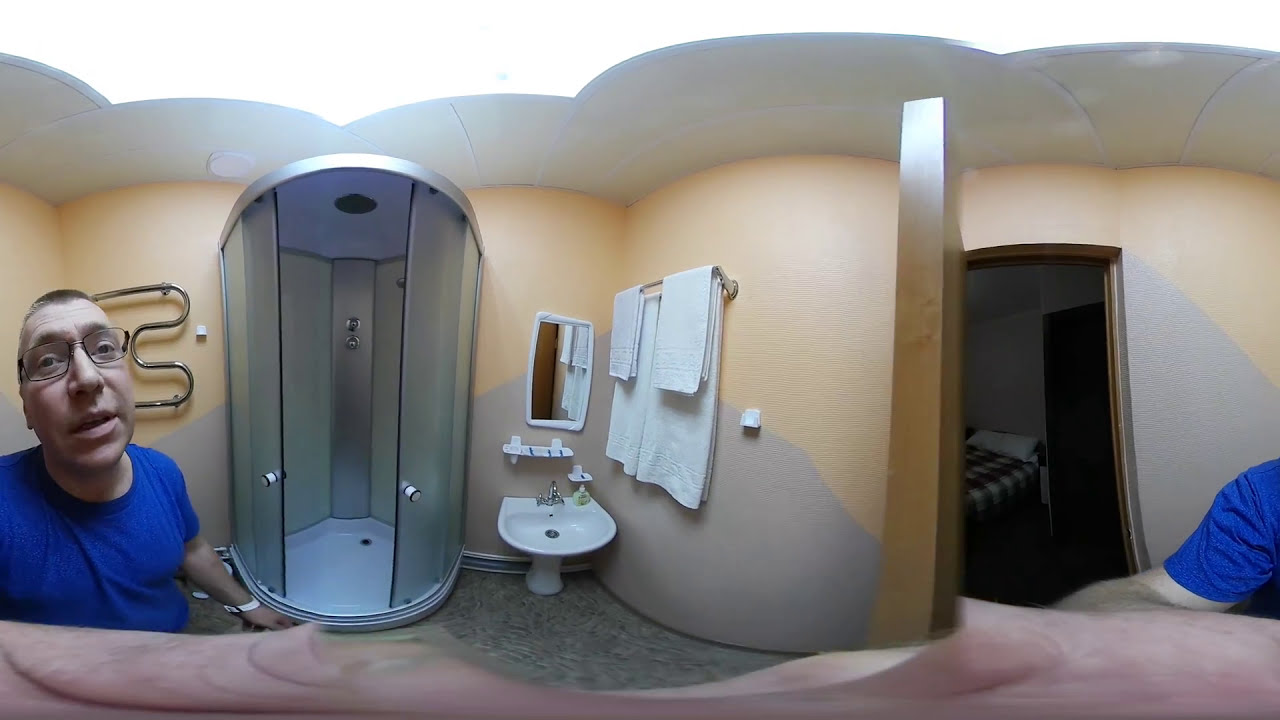In this distorted, fisheye-lens selfie, a middle-aged man with white skin, glasses, short-shaved hair, and a blue T-shirt is visible on both the left and right sides of the image due to the curved effect. He holds the camera with his left hand, which is adorned with a white watch. The bathroom setting includes a large stand-up shower with glass doors, a pedestal sink, and a mirror. On the right side, there are two white towels hanging from a curved towel hanger connected to the wall, and the walls are painted in cream and light purple. White light illuminates the scene from the ceiling. In the background, visible through a reflected doorway, is an adjacent dimly lit bedroom featuring a bed covered with a black and white bed sheet and white pillow covers.